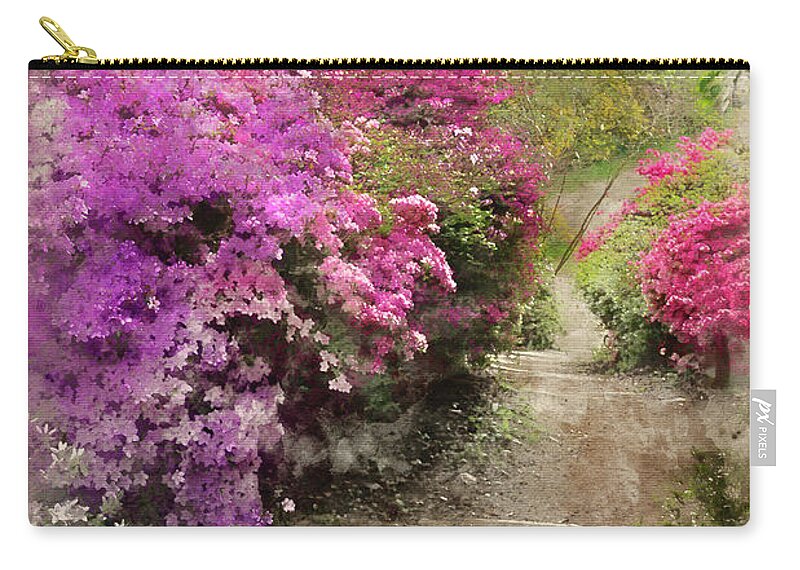This image captures a detailed product photograph of a cloth wallet or coin purse made from canvas-like material. The purse features a gold-colored zipper at the top, enhancing its elegant yet rustic appeal. The design on the coin purse serves as a key highlight, portraying a serene natural walkway likely within a forest or garden setting. This trail, seemingly made of dirt, meanders through vibrant shrubbery with blooming purple, pink, and white flowers on either side, suggesting a lush and healthy environment. The picturesque scenery is either a high-quality print or an iron-on design, epitomizing a tranquil hike through nature. Additionally, a small label on the side reads "PX Pixels," indicating the brand responsible for this uniquely artistic and functional accessory.